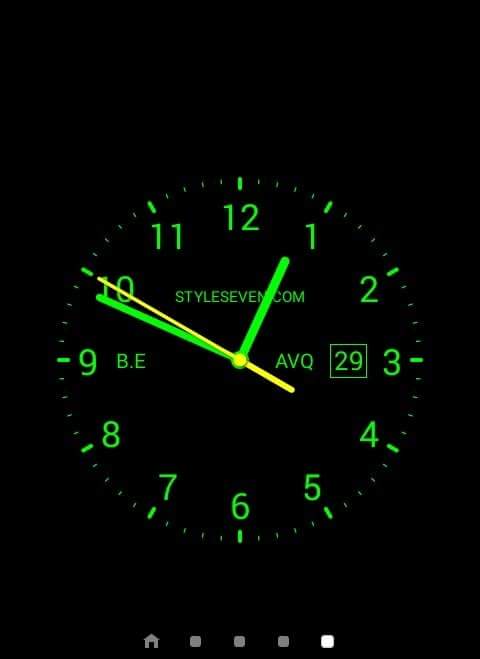The image displays a clock against a completely black background. The clock face consists of bright green neon numbers from 1 to 12, arranged in a circle. Surrounding the numbers, larger green dashes mark the hours, while smaller white dashes denote the minutes. The hour and minute hands are also green, while the second hand is yellow and pointed at the 10. The time appears to be 12:49. The clock is partially obscured by a green hour hand but shows the text "dial7.com" and "BE" near the 9 o'clock position, and "AVQ" near the 3 o'clock position. There's also a white-outlined box containing the green number "29" on the right. At the bottom of the image, there's a small icon of a house in green, followed by three grey squares and one white square on the right.